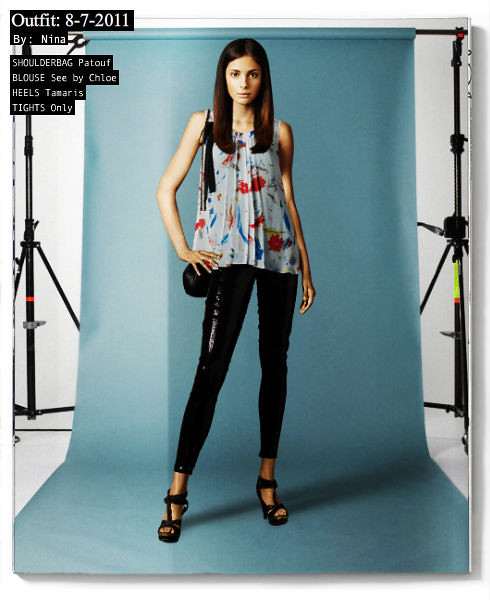A stunning photo captures a slender model with long brown hair cascading just below her shoulders, standing gracefully against a taut, teal-blue backdrop set up with supporting poles visible on either side. In the upper left corner of the image, white text on black bars reads: "Outfit 8-7-2011 by Nina," "shoulder bag, hat out," "blouse, See by Chloe," "heels, Tamaris," and "tights, Only." The model exudes confidence in a sleeveless, light blue floral-patterned blouse, paired with black, glossy leggings that stop just above her ankles, and stylish black high heels. One of her arms rests on her hip, enhancing her poised and professional demeanor, while the other hangs elegantly by her side. Her intense gaze is directed at the camera, though she remains unsmiling, adding to the seriousness and elegance of the shot.